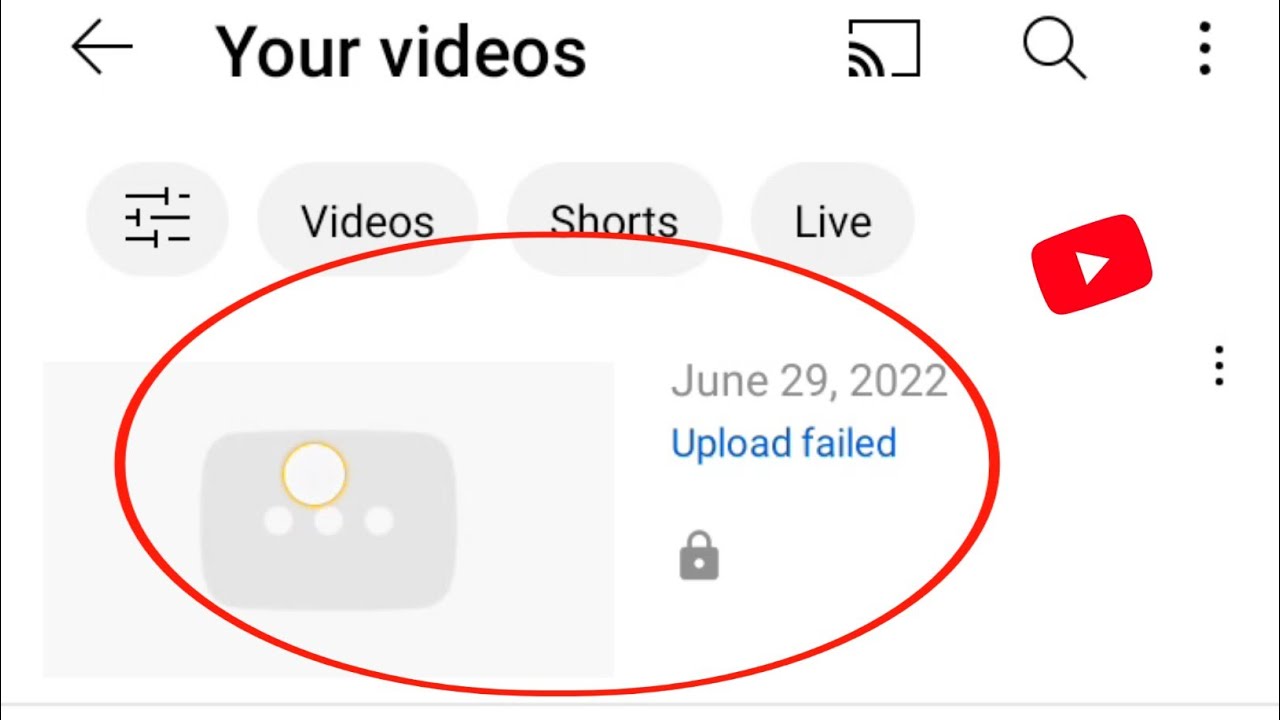The image features a simple YouTube interface on a white background, surrounded by a thin gray border. The top border is thinner compared to the more prominent gray lines running down the left and right sides. In the upper left corner, a bold black arrow points to the left, indicating a back navigation option. Next to the arrow, the phrase "Your Videos" is displayed in bold black font. To the right of this text, there is an icon resembling a screen share or Chromecast symbol, followed by a search icon, and a vertical three-dot icon, representing more options.

Below these elements, a filter option is visible, and the categories "Videos," "Shorts," and "Live" are listed. To the right of these categories is a red YouTube Play icon featuring a white play arrow in its center. A red circle is purposefully drawn around a specific section of the image, highlighting text that reads "June 29, 2022, Upload failed," accompanied by an unloaded profile image.

The overall layout suggests an issue with a video upload on YouTube, clearly marked by the red circle and associated with the date provided.